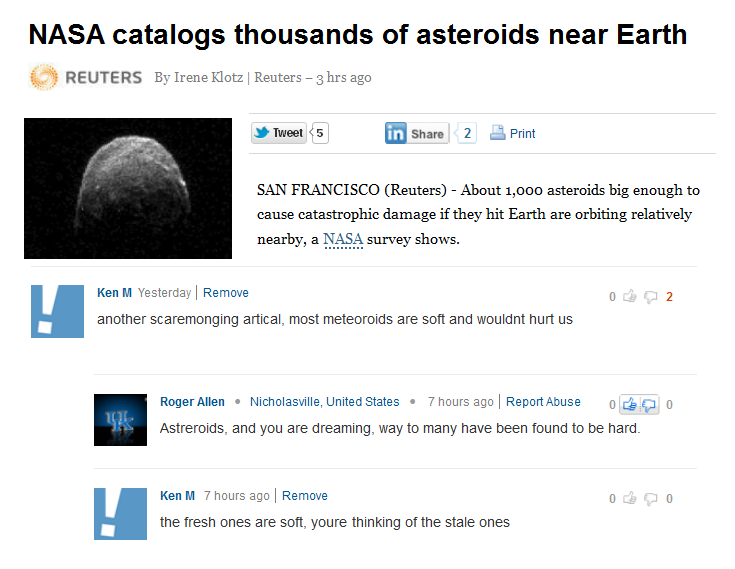This screenshot displays an article titled "NASA Catalogs Thousands of Asteroids Near Earth," authored by Irene Klotz for Reuters. The article was published three hours ago. It mentions that NASA has found 1,000 asteroids large enough to cause catastrophic damage, should they collide with Earth. This information is sourced from a survey. To the left of the text, there is an image of an asteroid set against a black background.

Above the article text, there are social media interaction buttons, including options to tweet, share, and print the article. Below the article, the comments section features a prominent discussion. 

The first comment is from a user named Ken M., posted yesterday, criticizing the article as "scaremongering" and claiming that most meteoroids are soft and wouldn't cause harm. This comment has received two thumbs down and no thumbs up.

Roger Allen responds, disagreeing and stating that many asteroids have been found to be hard. This comment has no likes or dislikes.

Ken M. replies, maintaining that fresh meteoroids are soft and the hard ones are stale. This reply also has no likes or dislikes.